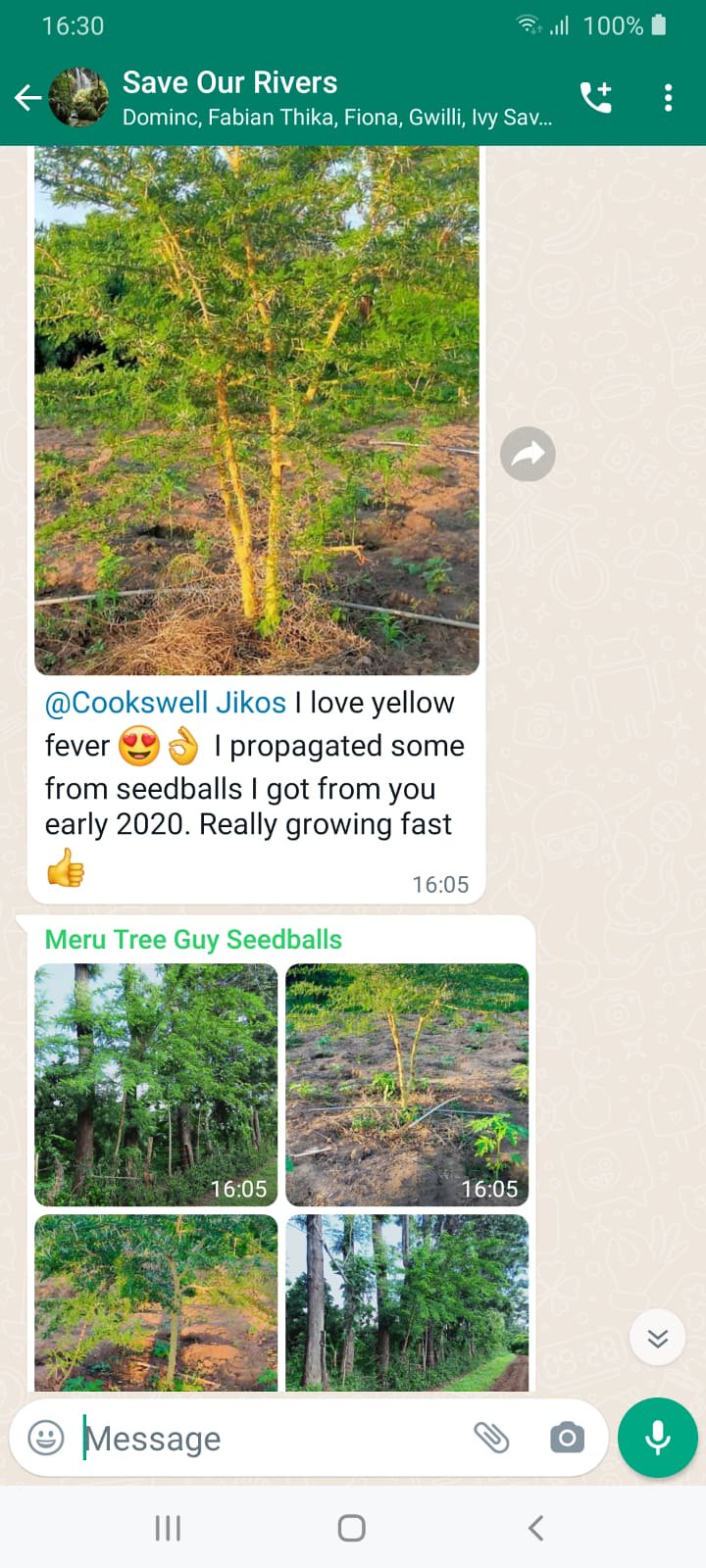A screenshot from a chatting app on a smartphone displays a conversation under a green header reading "Save Our Rivers" in white text. The participants, listed as Dominic, Fabian, Theka, Fiona, Gwily, Ivy, and Sav, discuss tree propagation. The topmost message features a large photo of a vibrant green tree with the caption: "Cooksville, Jicos (J-I-K-O-S). I love yellow fever. I propagated some from seed balls I got from you early 2020, really growing fast," followed by a thumbs-up emoji and a smiling face with heart eyes emoji. Below this, there is a series of four smaller images, credited to "MeruTreeGuySeedBalls." The four images depict various green trees: one showing a group of trees, another trees over a river, the third trees over brown soil, and the last depicting trees along a brown road. The interface includes a text bar for messages and a microphone icon in the bottom right corner.